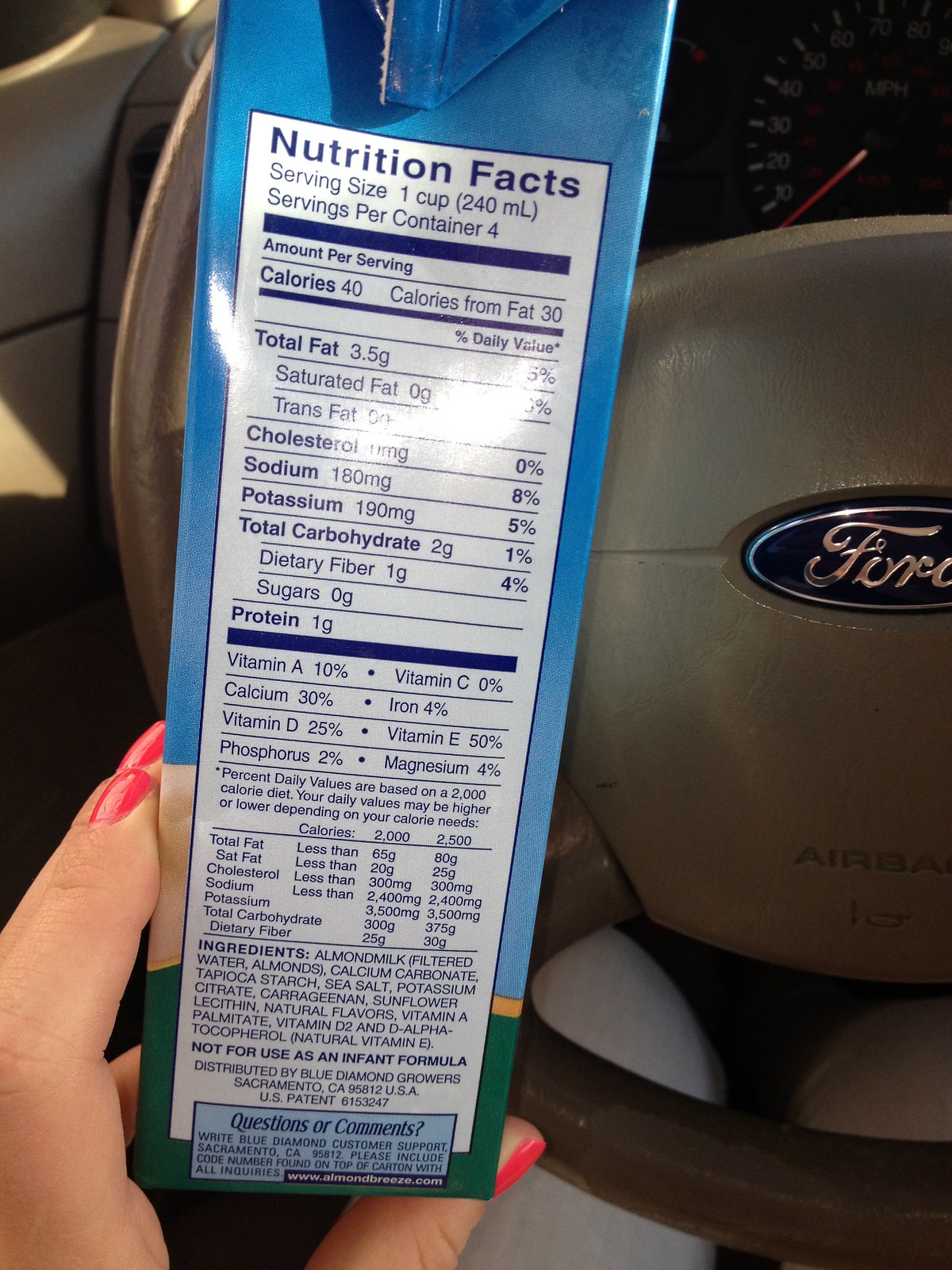The image is a vertically oriented portrait, approximately 75% taller than it is wide, featuring a person inside an automobile, holding up the side panel of a blue cardboard container, likely almond milk, revealing the nutrition label. 

The setting inside the car includes a visible segment of the steering wheel on the right side, prominently displaying the Ford logo. The logo is a wide, thin oval with a dark blue background, encircled by a silver border, with "Ford" elegantly written in silver cursive inside it. The "D" of "Ford" is slightly cut off by the image's edge. The steering wheel, composed of a dark leather-like material, continues down to the bottom of the photo but does not reach the far left edge. Only a partial segment of the wheel is visible, roughly 120 degrees of the full 360 degrees. The upper right corner of the image shows a hint of the speedometer, with its red needle pointing towards zero.

Central to the photo, slightly left of center, is the tall rectangular side panel of the cardboard food container, likely four to five times as tall as it is wide. The box has an unevenly folded top, resembling packaging typical of products like almond milk. The side panel primarily features a detailed nutrition label in dark blue ink. It starts with "Nutrition Facts" at the top, noting a serving size of one cup (240 milliliters) and four servings per container. Key nutritional information includes 40 calories per serving, with 30 calories from fat, 2 grams of total carbohydrates, 1 gram of protein, and vitamin content like Vitamin A at 10% and Calcium at 30%.

The ingredients list, near the bottom of the label, identifies the product as almond milk, listing its components as filtered water, almonds, calcium carbonate, tapioca starch, and more, all encoded in uppercase. The person holding the container is a woman, as indicated by her left hand, which is partially visible with her thumb and a couple of fingers adorned with bright, cheery red nail polish.